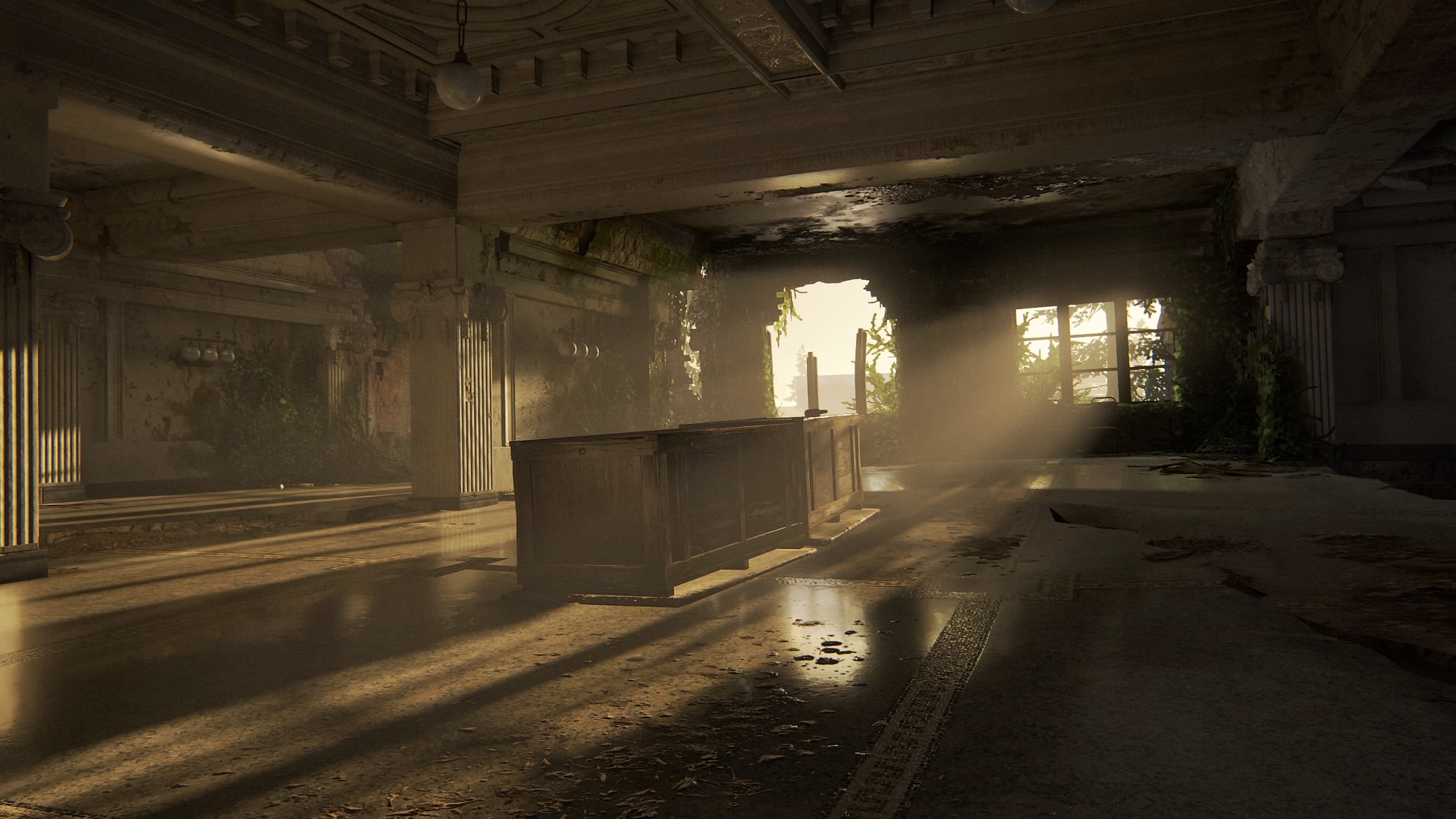The image appears to be a screenshot from a video game, depicting a dilapidated interior space. The scene is set in a broken-down building with significant water damage, evidenced by the rotten, ornate ceiling coffers. The central focus is a large, damaged wooden desk or cabinet. The floor is littered with grayish-brown, rough, and broken tiles. The background wall is partly destroyed, creating a jagged, rounded opening through which some foliage is visible, and there's a window to the right of this opening that allows bright sunlight to flood into the room. The left side of the image features a vine-covered wall and a view into a deeper part of the building, where columns and an additional opening can be seen. The overall atmosphere is dark, with light strips creating contrast, and the scene includes a wooden banister and perhaps a mirror, adding to the complexity and richness of the decayed environment.